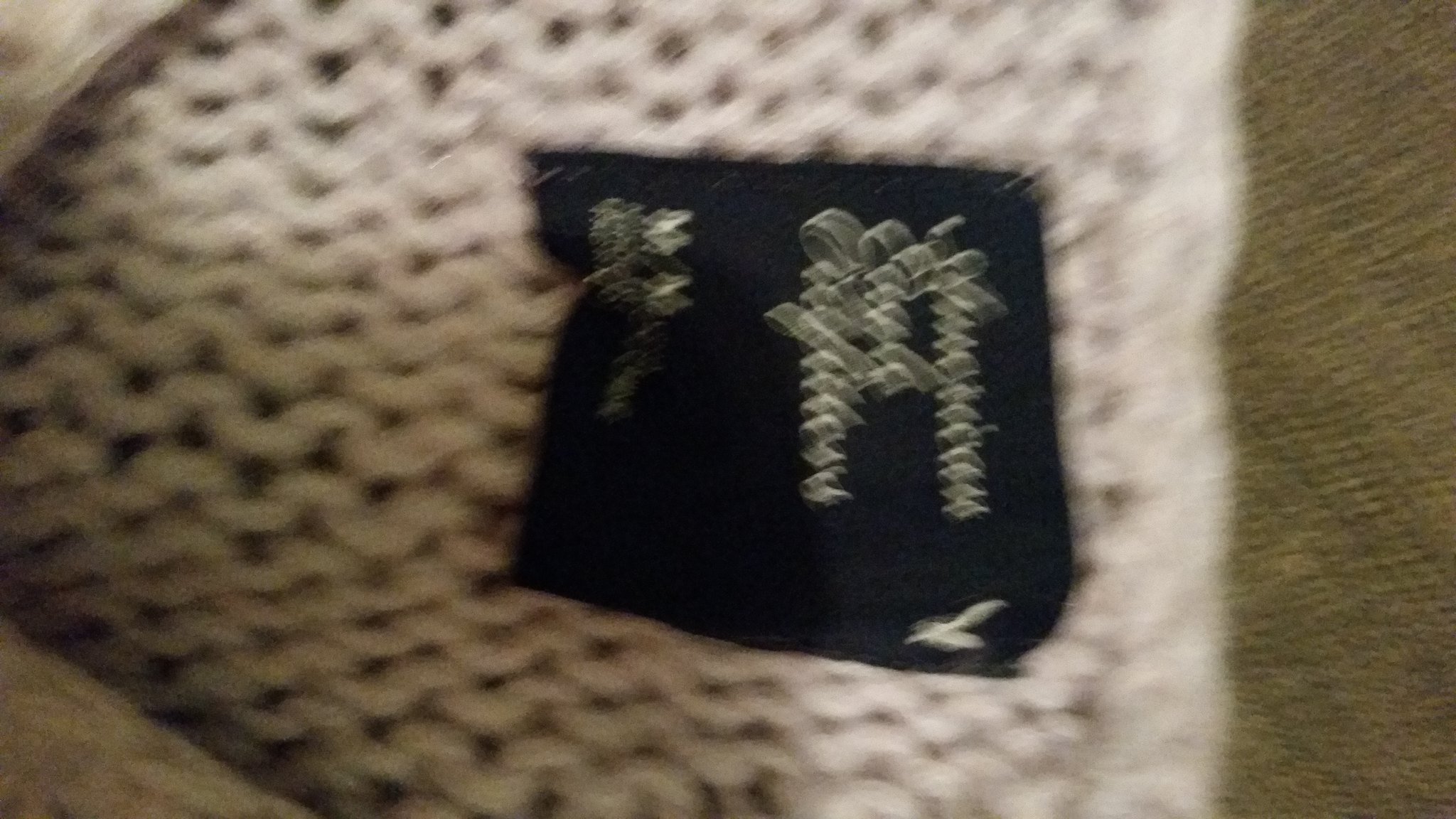The image is a very blurry close-up of a black square-shaped tag sewn onto a knit garment, possibly a shirt or a sweater, with intricate yarn stitches in a grayish cream or tan color. The background appears to be a greenish-brown surface, perhaps a carpet or a couch. On the tag, which is centrally featured in the image, there is unreadable cursive writing in a grayish silver or tan color. At the top right corner of the tag, there’s a logo resembling a bird, possibly an eagle. The overall blurriness makes it hard to discern specific details, but the tag seems to indicate the garment is a size medium.